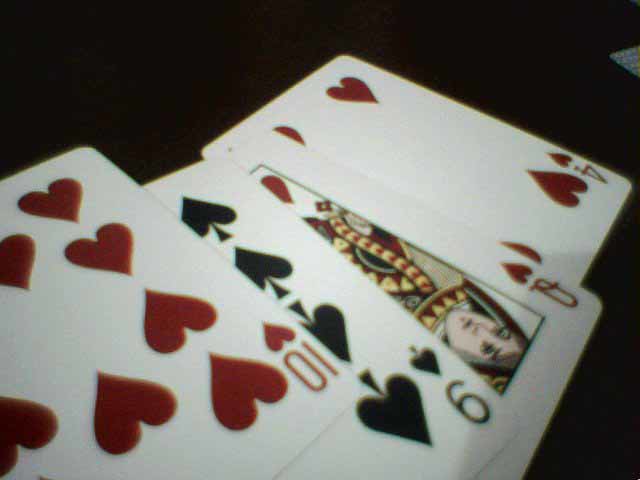This photograph, though slightly out of focus and appearing somewhat grainy, captures four playing cards arranged in an overlapping fashion on a dark surface that seems to be black or dark brown. The cards shown are the four of hearts, queen of hearts, nine of spades, and ten of hearts. The four of hearts is the most visible card, while the nine of spades is the most obscured but can still be seen surrounded by the queen and ten of hearts. The bright red and white colors of the hearts contrast with the black and white spades card. A noticeable reflection appears in the upper right corner, adding a touch of intrigue to the composition. A shadow cast over the cards suggests the photo was taken close-up or with a flash, contributing to the blurriness. Despite these imperfections, the distinct elements of the cards and their arrangement can still be identified.